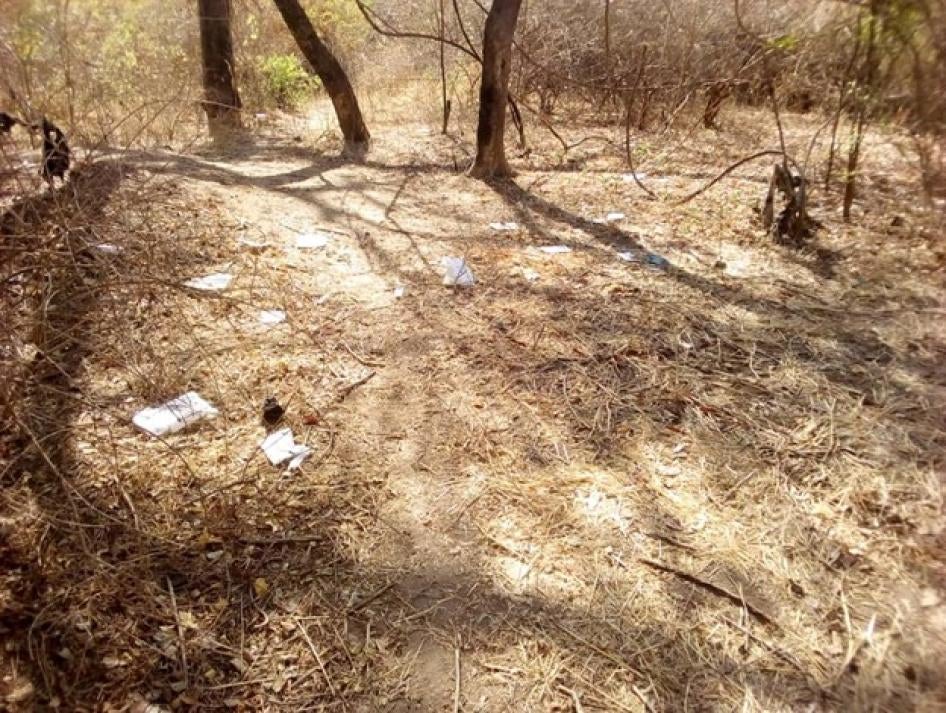This sepia-toned photograph captures a wooded area with a focus on the forest floor in the foreground. The ground is scattered with white litter, likely food packaging or tissues, suggesting human neglect. Dappled sunlight illuminates patches of the dry, grassy floor, creating a lighter appearance in some areas. Yellowish bushes can be seen towards the middle ground, adding to the autumnal feel of the setting. In the upper backdrop, three tree trunks stand prominently, with one leaning to the left, creating a rustic, somewhat deserted atmosphere. The branches are mostly barren, emphasizing the sparse and littered state of this outdoor space.